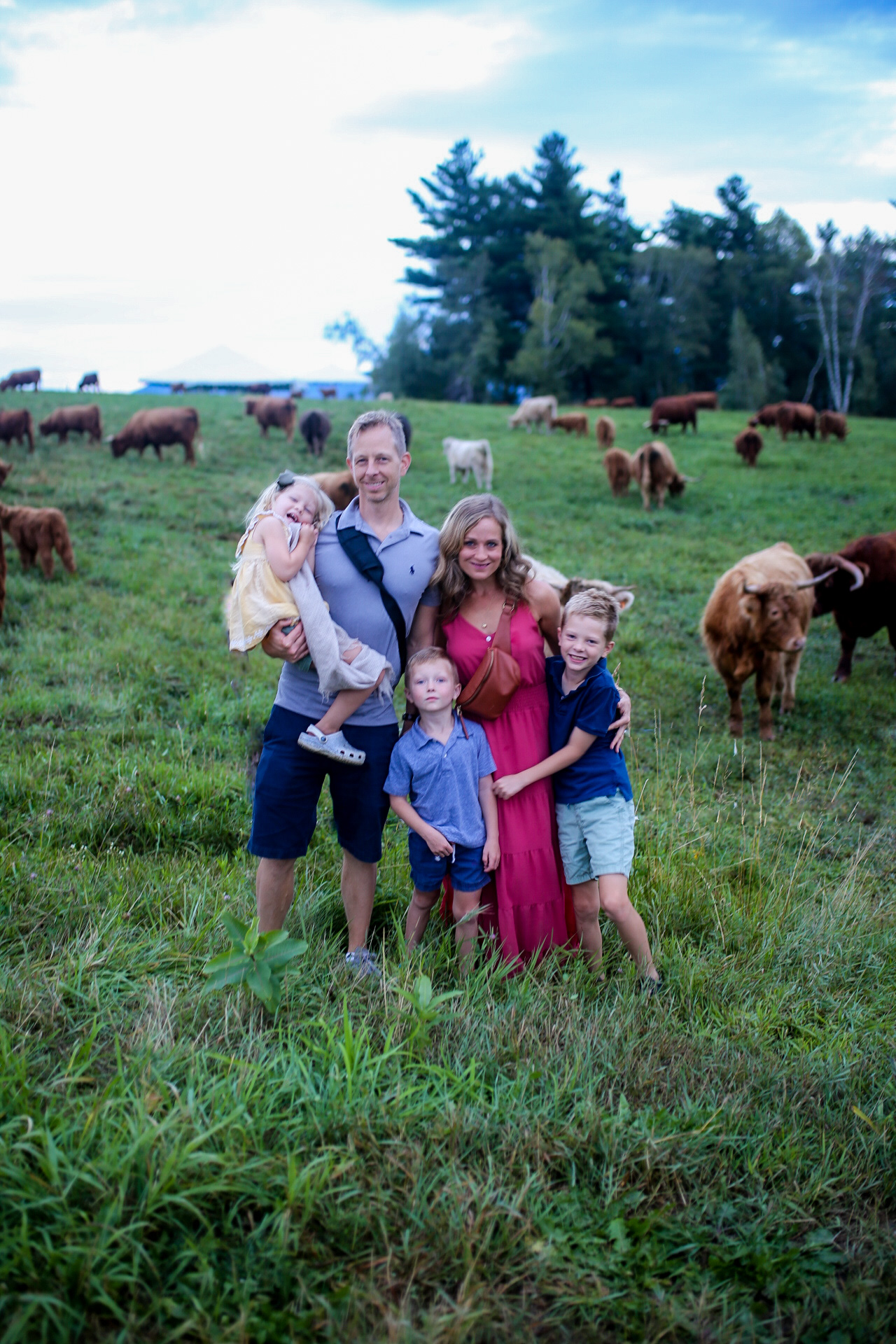In this idyllic family portrait set on what appears to be a farm, a family of five stands prominently in a vast, grassy field. The backdrop consists of numerous grazing cattle, predominantly brown with some white, many of which have long horns. Above, the sky is mostly clouded with patches of blue peeking through, framed by the lush trees further back. 

In the center, the father, dressed in a light purple polo and navy blue shorts, holds a smiling young girl about two years old, wearing a yellow and white dress and sporting blonde hair. He has a camera strap or backpack around him. To his right stands the mother, adorned in a long red (or fuchsia-colored) dress with long brown hair cascading down her shoulders. She carries a small purse over her shoulder and has her left arm around a boy, approximately 10 years old, in a blue shirt and blue shorts. Another boy, probably seven, stands close by, also in a blue shirt and shorts, with the mother’s right hand gently placed behind him.

Together, they form a close-knit and picturesque family, standing amidst the natural beauty of the field, surrounded by bovine companions and under a partially clouded sky.